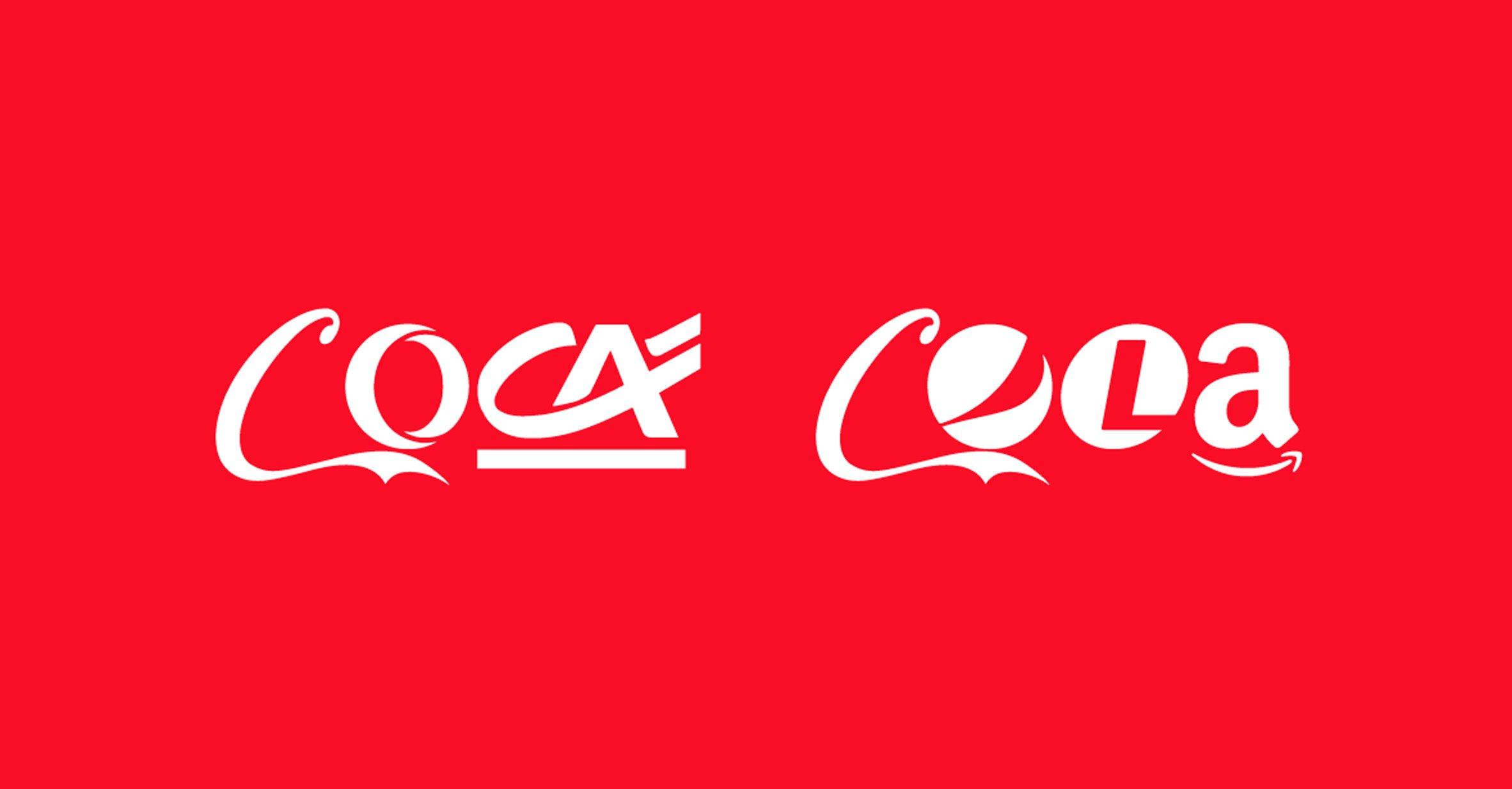The image features a horizontal red rectangle with a vibrant Coca-Cola red background, exuding a bright and eye-catching appeal. At the center, in white text, are the words "Coca-Cola," but unlike the classic Coca-Cola script, each letter is cleverly designed to resemble logos from various companies, creating a unique and playful typography. 

In "Coca," the first 'C' has an intriguing design, with the top resembling an alien antenna and the bottom mimicking a shark fin. The 'O' consists of two crescent moons facing each other, while the second 'C' looks like a delicate ribbon. The 'A' creatively overlaps with the preceding 'C' and is styled like a ribbon with an underscore beneath it.

In "Cola," the 'C' mirrors the first 'C' in "Coca," maintaining its alien antenna and shark fin style. The 'O' takes on the appearance of Pac-Man, distinguished by a leaf shape where the mouth is usually found. The 'L' is housed within a white circle, and inside it is a red 'L,' emphasizing the Coca-Cola theme. Finally, the 'A' is reminiscent of the Amazon logo, complete with the characteristic smiley arrow underneath.

This inventive restyling maintains the recognizable red and white color scheme of Coca-Cola while showcasing an imaginative blend of various logo-inspired letters.